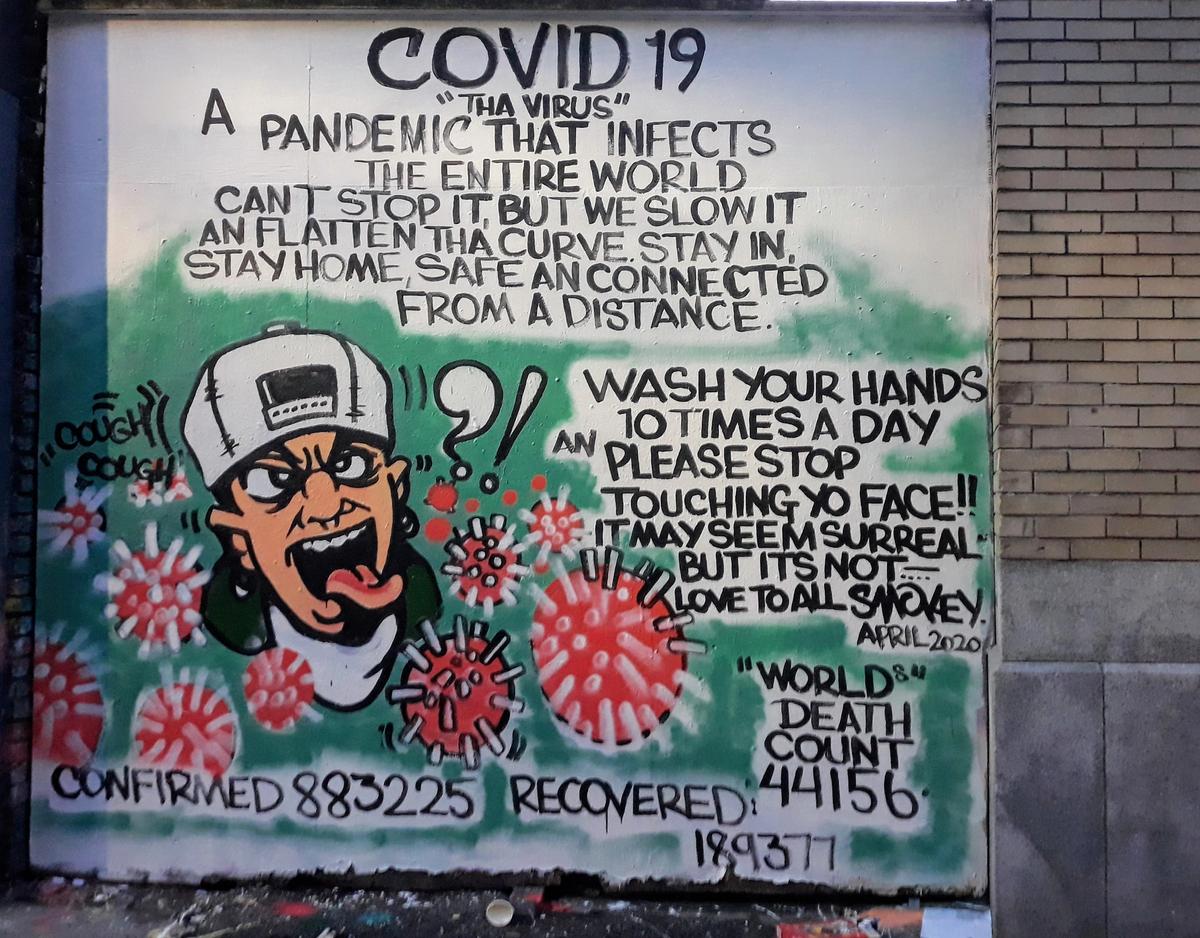This outdoor photograph captures a detailed wall mural set against a background of brick and concrete. The mural is primarily white, featuring bold black capital letters at the top reading "COVID-19" and, in quotes, "the virus." Below this, it states: "A pandemic that infects the entire world. Can't stop it, but we slow it and flatten the curve. Stay in, stay home, stay safe and connected from a distance." On the lower left side, there is an image of a cartoon character with a backwards white cap and his tongue sticking out, surrounded by red circles representing the coronavirus. Text near him includes "cough, cough." To the right of the character, the mural instructs: "Wash your hands 10 times a day and please stop touching your face. It may seem surreal, but it's not. Love to all. Smoky. April 2020." Additionally, the mural provides daunting statistics: "World death count 44,156. Confirmed 883,225. Recovered 18,189,377." This vivid artwork delivers a powerful and urgent message to remain vigilant against COVID-19.